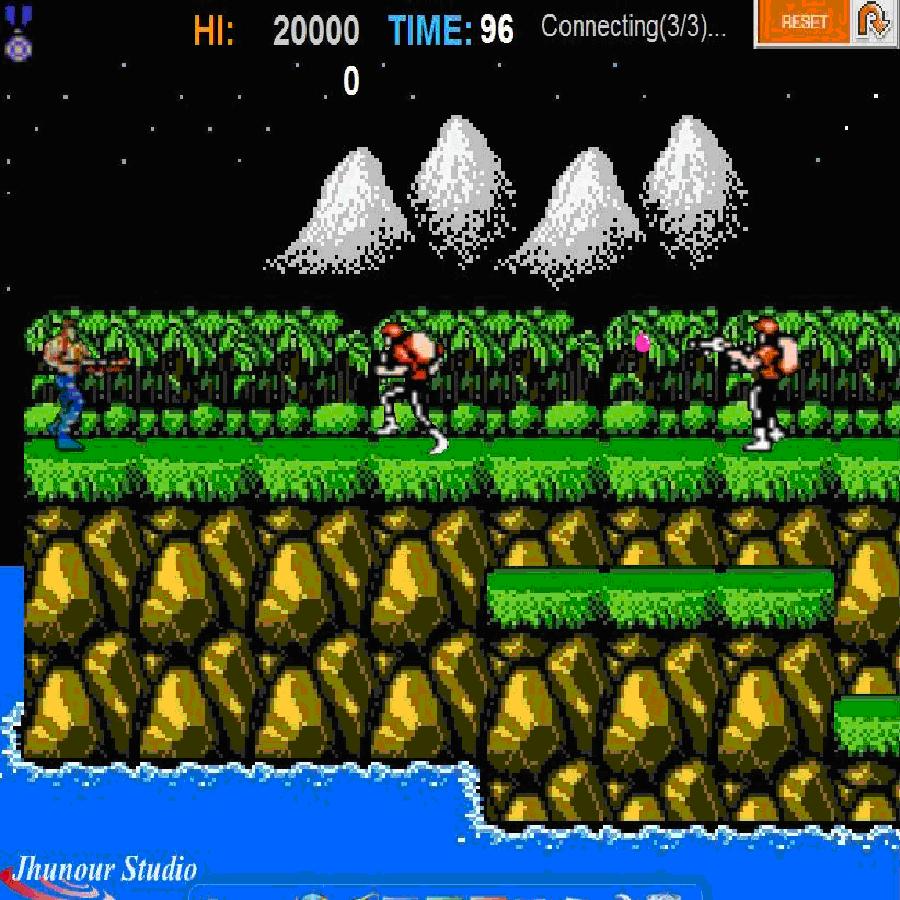The screenshot depicts an old video game with a square screen, featuring distinct visual elements and multiple levels of terrain. The top third of the screen has a black background, dotted with white stars, evoking a starry night sky. Across the very top, there's text that reads "H-I-N" in orange blot print, "2000" in white, "time" in blue, "96" in white, and "connected," reminiscent of a modem connection display. In the upper right corner, there's an orange reset button with a small arrow circling around it.

The central part of the screen shows a green area with land and trees, resembling a cliffside with three distinct flat surfaces arranged in different levels. On the highest level, three figures are engaged in combat. The figure on the left, wearing blue pants and a red plaid shirt, appears to be holding a gun. The other two figures, one in a red jacket or backpack and the other with a similar red top and something on his back, are positioned centrally and to the right, both seemingly in motion towards the left figure. The middle character is shooting, indicated by a pink projectile emitting from his gun.

Below this central combat scene, there are stylized rocks leading down to a lower level of flat ground, and finally, a blue body of water at the bottom of the screen. In the lower left corner, a caption reads "G-H-U-N-O-U-R studio" against a green background with a red concentric circle swirl, highlighting the game's developer.